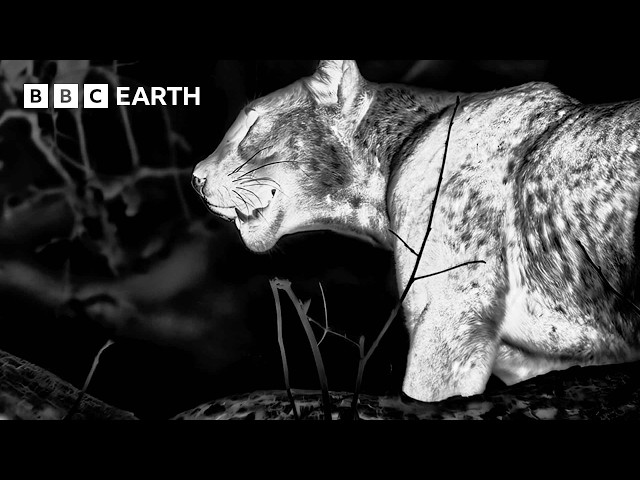This black and white image, taken from a BBC Earth documentary, showcases a high-contrast, night vision or heat vision scene. The central focus of the photo is a large, spotted jungle cat, likely a leopard, jaguar, or cheetah, with only its head and front torso visible. It has a bright white appearance with smaller dark gray and black spots, indicating the use of specialized camera mode. The cat’s mouth is open, giving an impression of surprise or mid-hunt activity. Overlaid in the foreground and background are indistinct branches and leaves, contributing to the jungle or forest setting. The top left corner features the BBC Earth logo in white font. The vivid contrast and intense coloring suggest a visually striking and detailed capture of the cat in its natural nighttime environment.